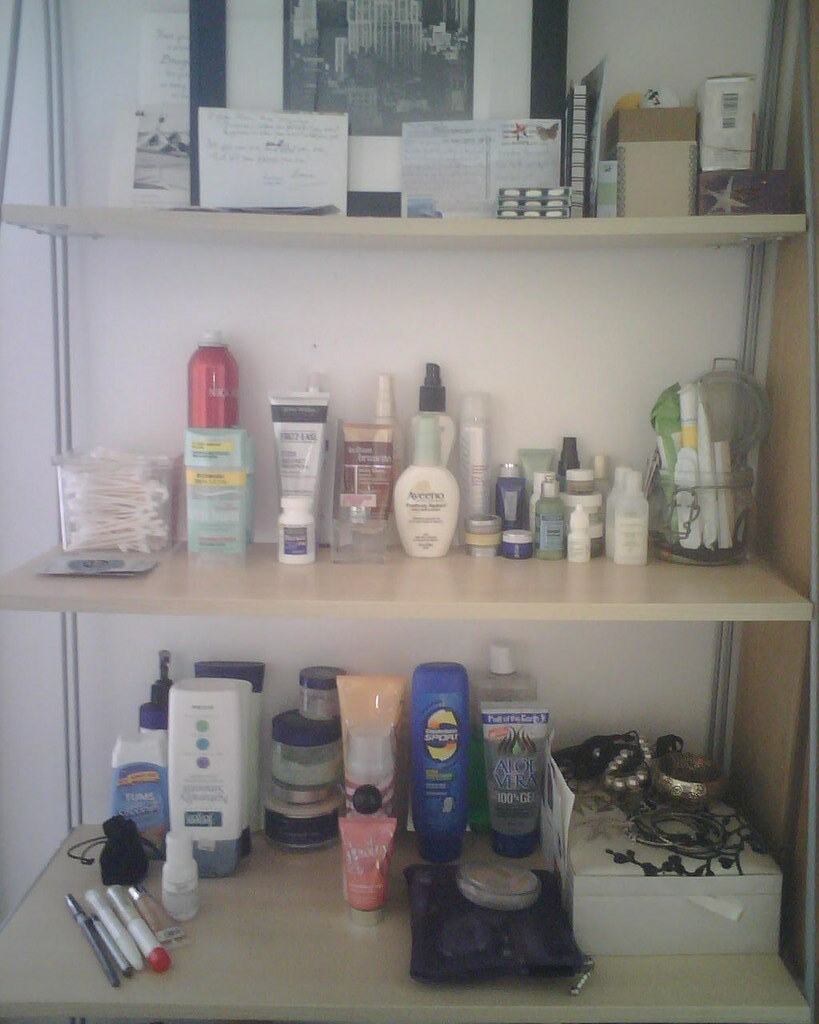This image showcases a neatly organized set of shelves, likely located in a room or closet, each adorned with a variety of items. The top shelf features a framed picture alongside various gadgets. The middle shelf appears to be dedicated to cosmetics, displaying a bottle of Avino lotion, a container of Q-tips, and several jars and bottles of assorted beauty products. The bottom shelf holds what seems to be jewelry on top of a white box, a bottle of suntan lotion—possibly Coppertone—and facial wipes, interspersed with more jars and bottles. The shelves themselves are of a muted tone, contrasting with the vividly colored items in shades of blue, red, green, orange, white, and black. The white wall behind further accentuates the colorful and diverse assortment of neatly arranged products, making the entire setup visually appealing.